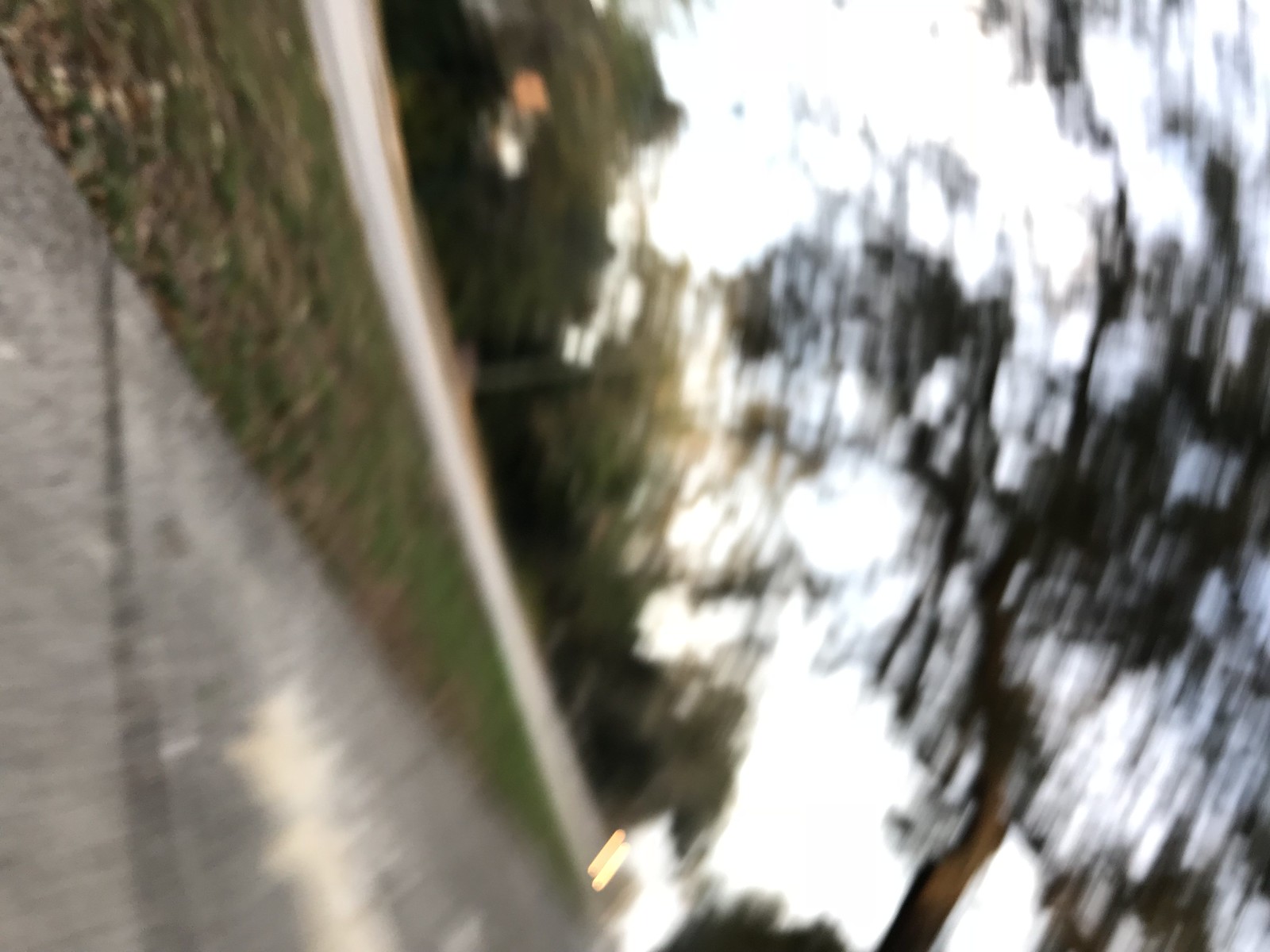This blurry, out-of-focus outdoor photograph, currently positioned sideways, depicts a scene that if rotated a quarter turn clockwise would appear correctly oriented. In the bottom left corner and extending down most of the left side, a gray sidewalk is visible, identified by a black expansion joint running vertically. Above this sidewalk in the left corner, a patch of grass stretches toward the middle of the bottom edge, spotted with patches of white and brown amidst the green.

Adjacent to the grass, a strip of white indicates a roadway. Beyond this, the scene is filled with an array of trees and bushes. A lighter area suggests the presence of a house window, though the house itself is not clearly visible. The right side of the image is dominated by the sky, with a tree branch emerging from the bottom right corner and dark leaves hanging over the sidewalk. Near the bottom of the image, just to the left of the center, two yellow streaks likely represent headlights.